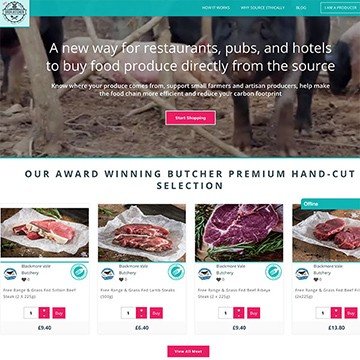This image features a turquoise-colored border at the top, accompanied by slightly blurry text. The main visual depicts a traditional pigpen with two pigs, one pink and one black, lying on the ground. The text overlay reads: "A new way for restaurants, pubs, and hotels to buy food produce directly from the source. Know where your produce comes from, support small farmers and artisan producers, help make the food chain more efficient, and reduce your carbon footprint." Below this text is a pink rectangle, presumably a clickable button, although the text on it is not visible. 

Further down, additional text promotes "our award-winning butcher's premium hand-cut selection," displayed alongside four images of steaks. Each steak image includes heart ratings, some sort of seal or stamp, and descriptive text within a white box, flanked by two pink boxes, with a number placed at the bottom.